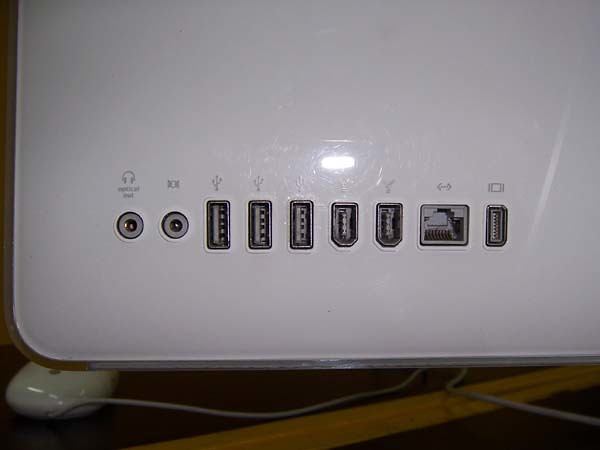This color snapshot, horizontal and rectangular in shape, showcases the back of a vintage Apple computer or monitor. The white plastic surface, taking up most of the frame, has a slight sheen and is set against a dark wood desk trimmed in light wood. The focus of the image is on the numerous ports lined up from left to right along the bottom edge of the device. Starting from the left, there are two headphone jack-like ports, followed by three USB ports with visible USB logos above them. Next are two FireWire ports, identifiable by their rectangular tops and beveled edges, and an Ethernet port marked by a unique logo featuring two arrows and dots in the center. Lastly, there is a video jack port, recognizable by a square with two vertical lines next to it. A classic wired Apple mouse with a grey cord and white oval body, adorned with a grey Apple logo, can be seen partially under the device. The image is taken indoors with a flash illuminating the details of the ports and the surrounding setup.